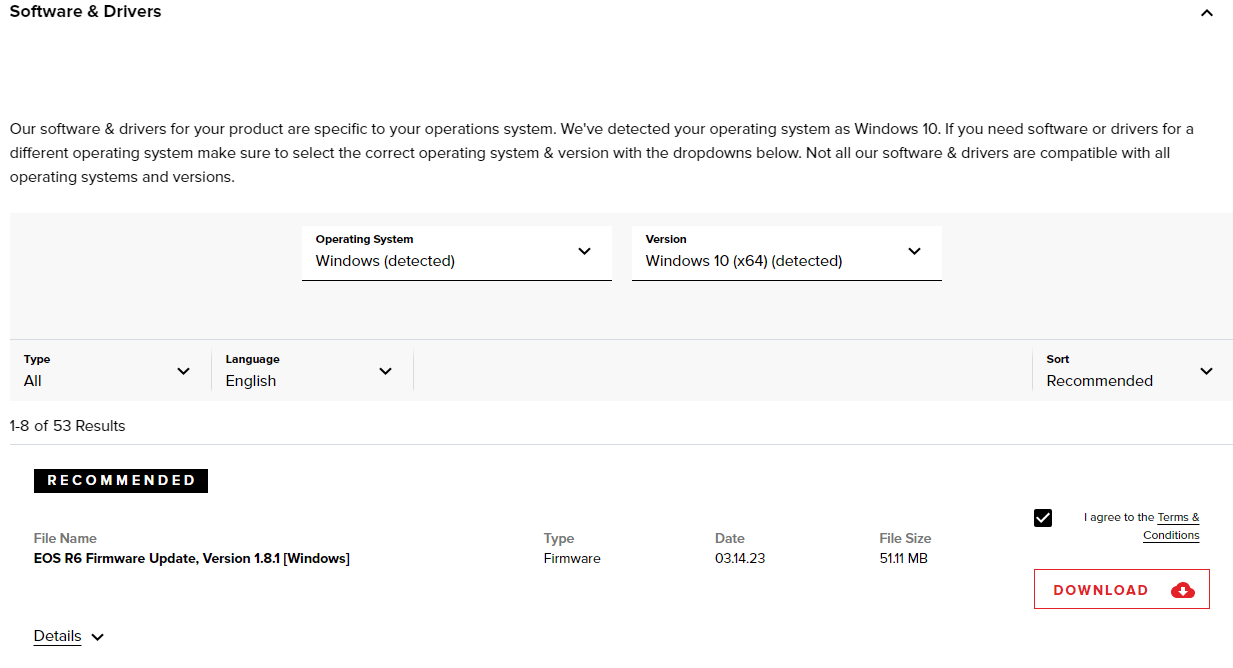The image, titled "Software and Drivers," features a clean white background. In the upper left-hand corner, the phrase "software and drivers" is displayed in black font. On the upper right-hand corner, a black upward arrow is visible. Below the arrow, there is a paragraph of text explaining that the software and drivers shown are specific to the detected operating system, which is identified as Windows 10. The paragraph emphasizes the importance of selecting the correct operating system and version from the dropdown menus below, as not all software and drivers are compatible with every operating system and version. Further down, two dropdown options are presented. The first dropdown is labeled "Operating System" and indicates "Windows" as detected. To the right of it, another dropdown labeled "Versions" displays "Windows 10."